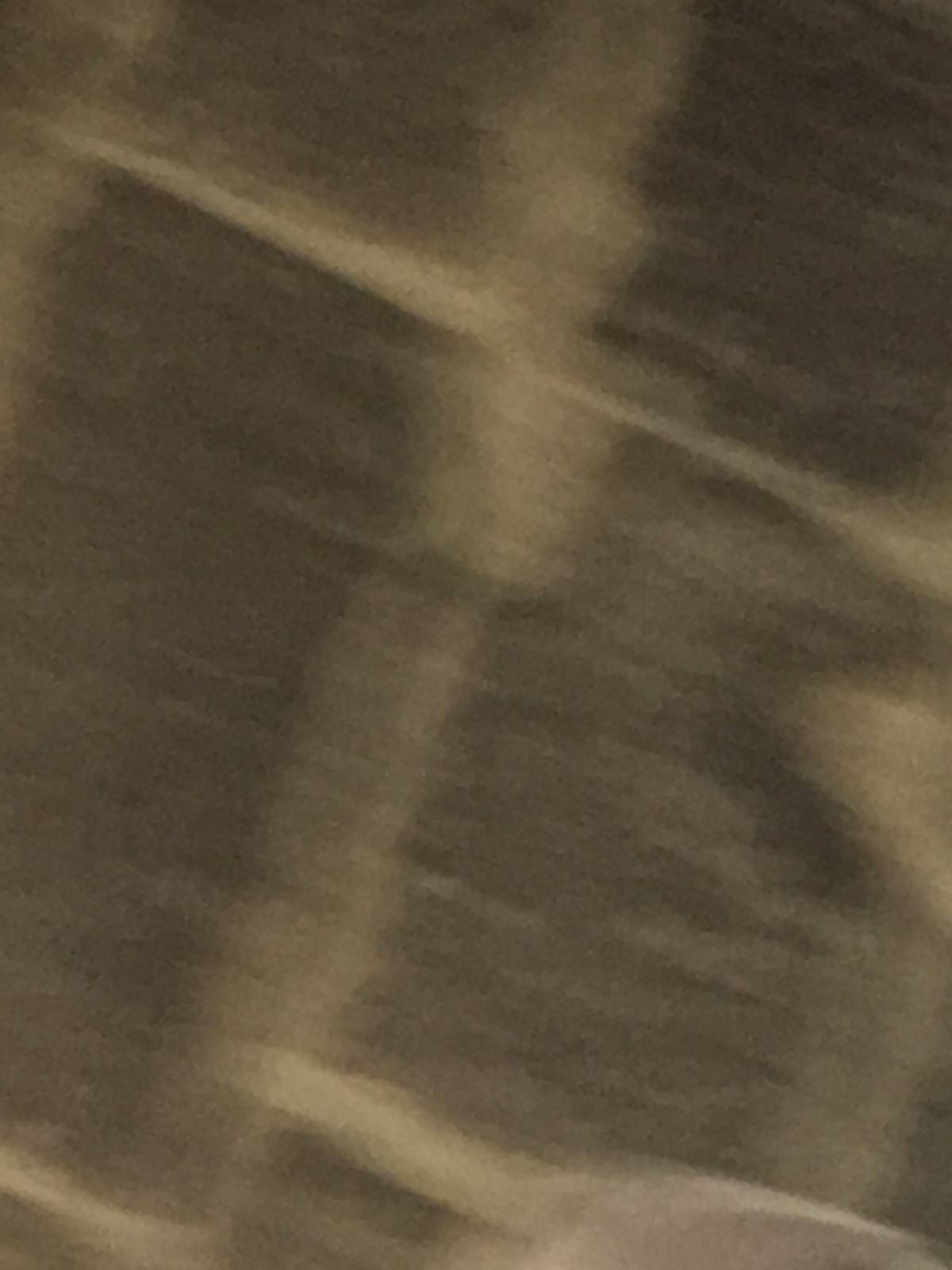The photograph seems to be intentionally blurred, featuring a palette dominated by shades of tan and grayish brown. The lower left corner showcases a distinct, straight area of brown, intersected by a pale beige line that extends upward. Approximately a few inches from the bottom, this pale beige line broadens into a larger, light beige blob. A horizontally tilted line intersects this blob and stretches toward the top of the photograph, flanked by darker brown areas on either side. The right-hand corner also contains patches of beige-ish brown. The overall composition and blurriness suggest that this might be an abstract or unfocused image of a window pane.